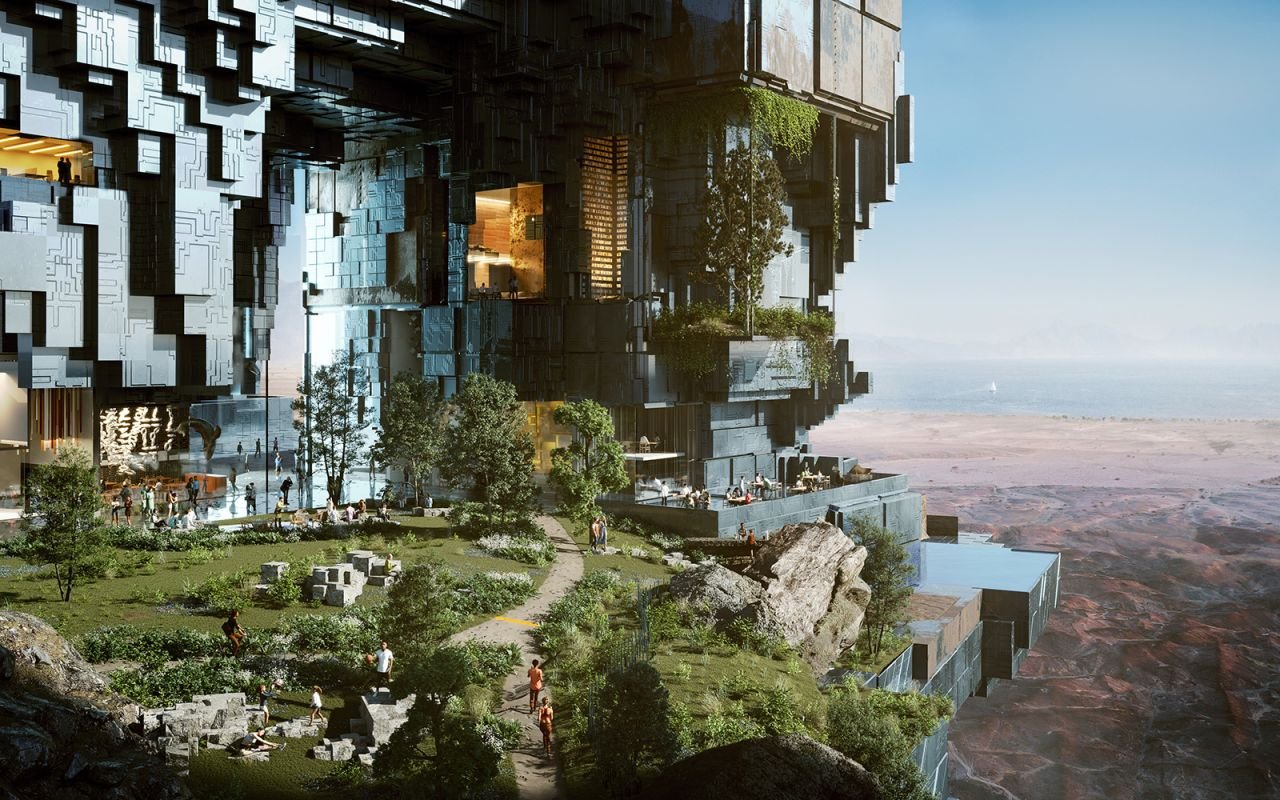This evocative, computer-generated artwork depicts a large, futuristic structure perched precariously on the edge of a precipice, overlooking a vast, scenic valley. The imposing building, reminiscent of a computer diagram or a mosaic of metal cubes, features numerous reflective glass surfaces that capture and mirror the blue sky above. It is adorned with greenery, including trees and bushes, some of which dangle off the sides, adding a touch of nature to the modernist design.

In the foreground, there's a lush grassy area with a path running through it, where several people are seen walking, jogging, or riding bicycles. The grassy section also features vibrant human activities, such as kids playing basketball and people enjoying a picnic or dining on a patio equipped with tables. The setting is outdoors with an array of rich colors that enhance the depth and detail of the image.

Beyond the building, the landscape stretches into a breathtaking view where the rugged terrain transitions into a desert plain. In the distance to the right, one can spot a serene body of water, possibly an ocean, with a small ship sailing far off. The overall composition of this image gives a sense of immense height and infinite expanse, blending futuristic architecture with natural beauty in a harmonious balance.